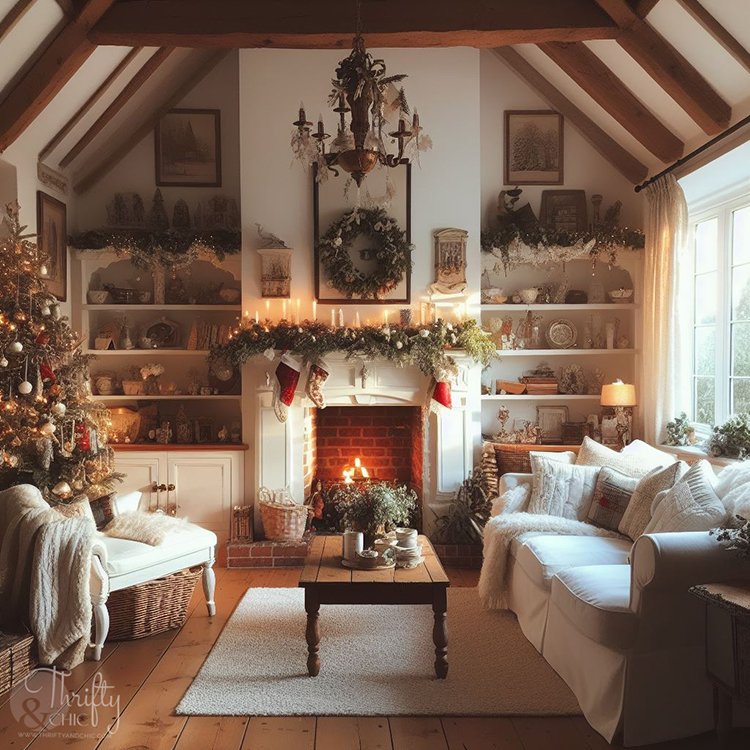This photograph captures a cozy and elegantly decorated living room set perfectly for the holidays. Central to the composition is a white fireplace, complete with a white mantle that reaches up the back wall, adorned with stockings, lit tapered candles, and lush greenery garland. Above the mantle, a vibrant green wreath with decorative accents adds festive charm. The fireplace has a brick back wall and warmly lit candles inside, contributing to the room's glowing atmosphere. 

To the left of the fireplace stands a fully decorated Christmas tree, featuring gold lights, white baubles, and possibly red bows. The back wall is lined with bookshelves, enhancing the homely yet stylish feel of the space.

On the right side of the room, a white cotton sofa is laden with fluffy white pillows and blankets, facing a window that lets in natural light. Directly in front of the fireplace, a wooden coffee table rests on a white, fluffy area rug, adding to the comfortable ambiance. To the left side of the coffee table, there's a cozy chaise lounge, also in white, with a blanket and pillows, inviting relaxation.

The hardwood floors and the ceiling, which features contrasting brown wood beams against a white background, complete this warm and homey living room scene. The entire setup exudes an air of welcoming elegance, perfect for the holiday season.